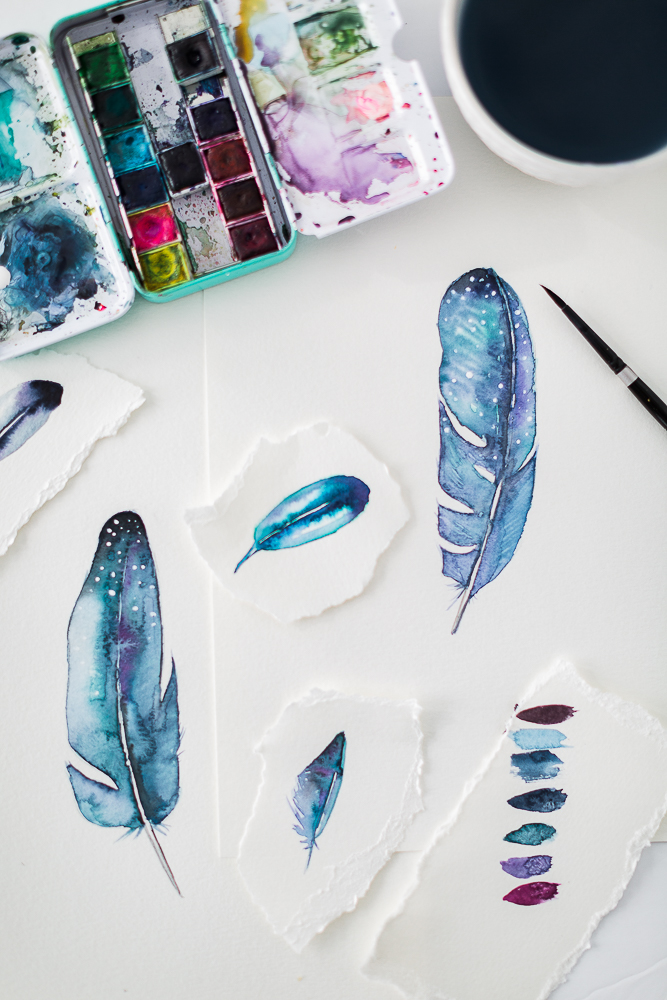The image shows a rectangular workspace, taller than it is wide, depicting an art project in progress on a white table. In the center, there are several detailed paintings of feathers, primarily in light blue and purple hues with intricate white lines, slits, and dots. These art pieces are on both large and torn pieces of white paper. To the bottom right, a piece of torn paper serves as a color key, featuring neat rows of seven different paint samples in a variety of colors including browns, blues, greens, purples, and reds. The workspace is quite messy; an open tin of children's paints sits at the top with blotches of paint splattered across its surface, encasing rows of small paint squares. In the top right corner, a white cup filled with a dark liquid, possibly black coffee or water for cleaning brushes, is present. Below it lies a black pen with a silver stripe wrapping around it, its pointed end emerging from underneath. A paintbrush's tip also protrudes from the right-hand side of the image, contributing to the overall scene of creative activity and organized chaos.